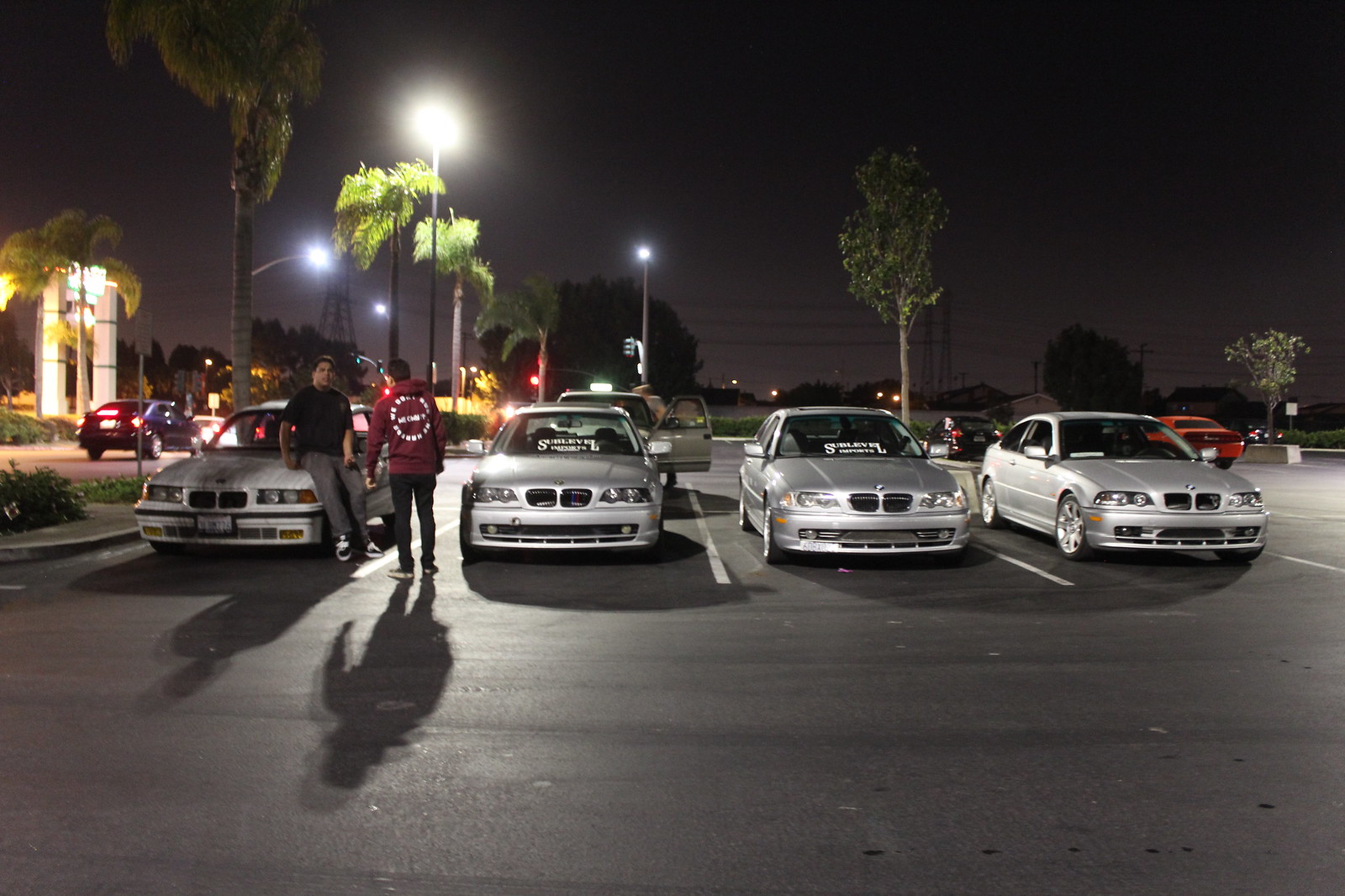In the dimly lit evening parking lot, four identical silver BMW cars are lined up in a row, facing the camera. The parking lot is illuminated by tall street lights, with four visible lights casting a glow over the scene. Beyond the neatly parked BMWs, more vehicles are scattered throughout the lot, including one directly behind the second BMW with its door ajar, indicating someone is entering or exiting. Two men are positioned between the first and second BMWs. The man on the left is casually seated on the hood of the first car, dressed in a black shirt and grey pants, exuding a relaxed demeanor. Beside him, the other man stands in a red hoodie with white writing on the back, engaging in conversation. Surrounding the parking lot are various trees, including distinctive palm trees, suggesting a warm, tropical climate. To the left of the lot, a building with lit windows can be seen, adding to the background of the bustling scene. Additionally, a road runs nearby on the left side, with a couple of cars currently driving along it, their red lights visible in the distance. The parking lot appears lively, juxtaposing the calm of the parked BMWs with the motion of incoming and outgoing cars.